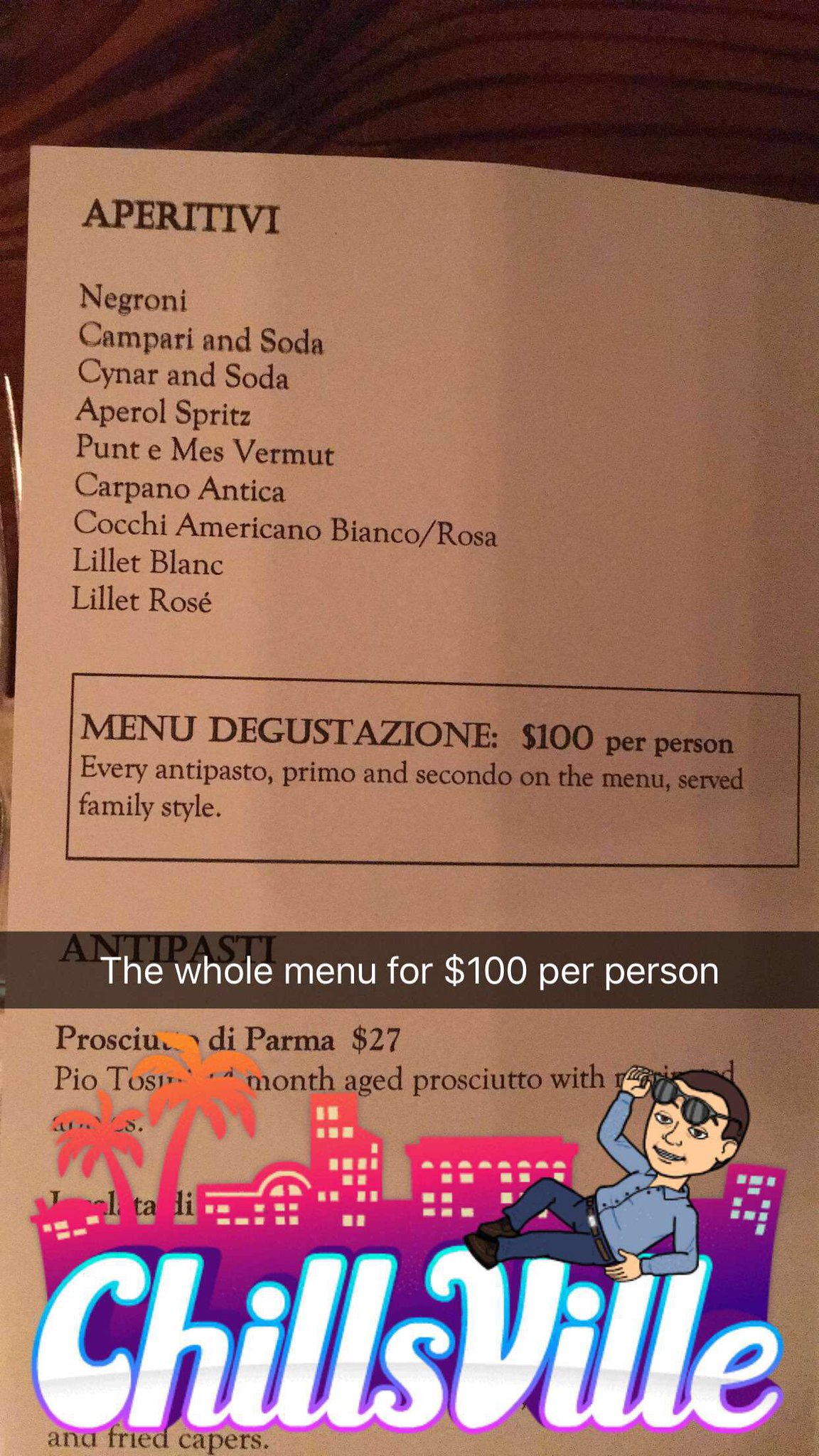The image prominently features a stylish and modern menu, centered as the focal point. Towards the lower part of the menu, there is a semi-transparent black block with white lettering advertising "The whole menu for $100 per person." The menu itself includes a variety of text, including dish names that appear to be in French, indicating a diverse culinary offering, alongside numerous English descriptions.

At the bottom of the image, there's a creatively designed graphic with the phrase “Chillsville” in white letters, each with a colorful border gradient that shifts from teal to blue to purple. A small character is seen seated atop the letters to the upper right, adding a playful touch. An illustrated city skyline can be seen in the background featuring two palm trees on the left, with the sky transitioning from neon pink to a medium orange hue, evoking a vibrant sunset.

The entire menu is laid upon a well-finished, varnished wooden surface, lending a warm and inviting background to the composition.